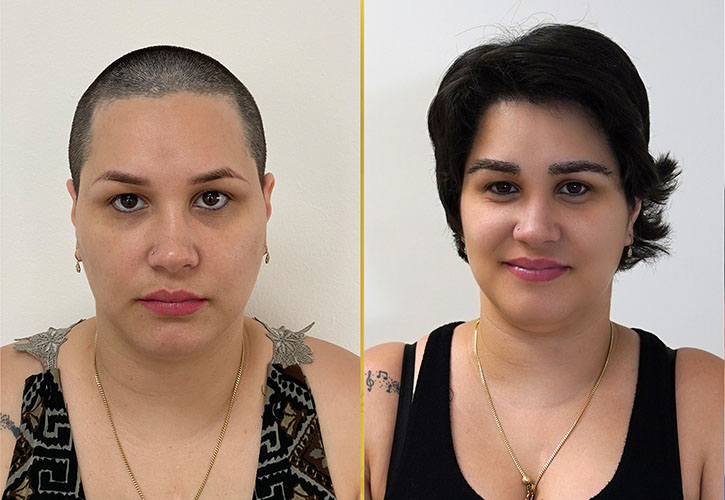The image juxtaposes two photographs of the same woman, presented side-by-side to highlight a transformation in her appearance. In the left photograph, the woman has a medium-dark complexion and sports a very short, shaved hairstyle. She is adorned with small earrings and a gold necklace, partially obscured by the straps of a black patterned garment—possibly a shirt or dress. In contrast, the right photograph showcases the woman with a medium-length, thick hairstyle. Despite the change in hair length, she retains her gold necklace, though the design specifics are indistinct. Her attire also shifts to a simple black tank top. The image contains no text, focusing solely on the visual transformation.